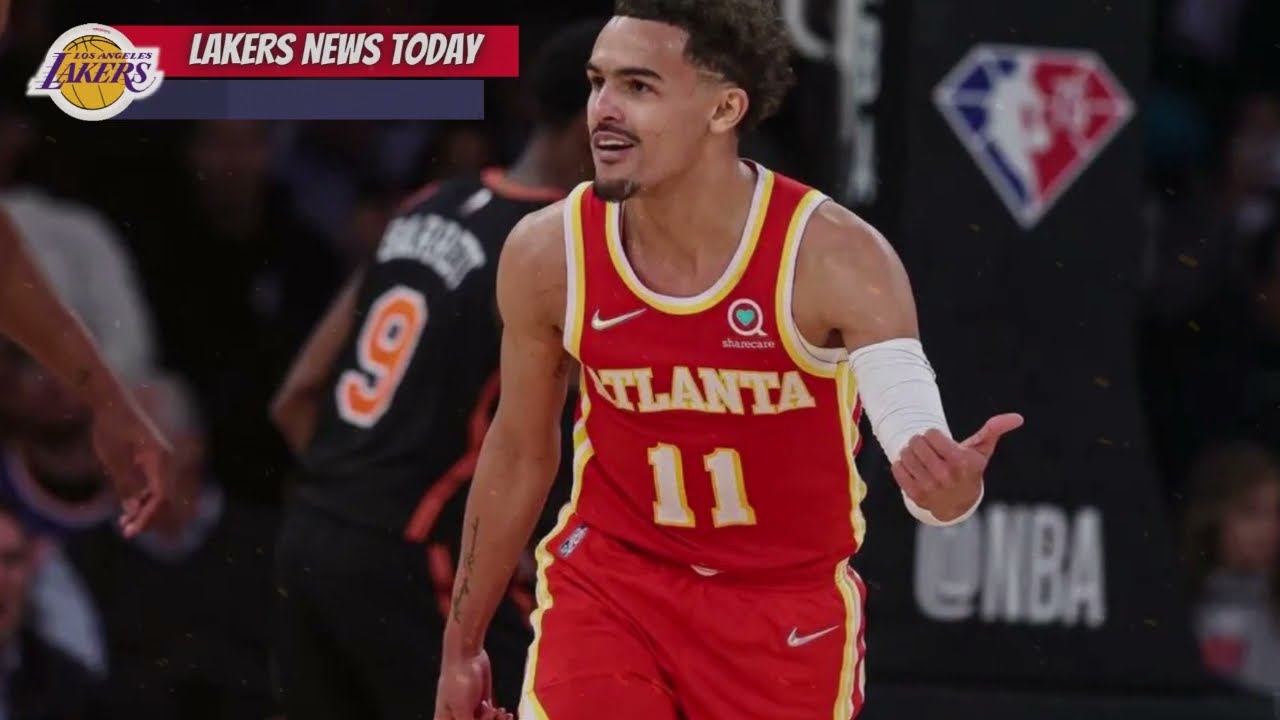The image is a detailed screenshot from a basketball game between the Los Angeles Lakers and the Atlanta Hawks. Front and center is basketball player Trae Young, identified by his distinctive black hair, goatee, and mustache. He is sporting a red Atlanta Hawks uniform, which features the name "Atlanta" and the number "11" in white and yellow on the front. His uniform is adorned with yellow and white stripes along the edges. Young has a white bandage wrapped around his forearm and bicep, and he is making a pointing gesture with his left hand, his thumb directing towards the left. 

To the left side of the image, in the upper corner, there is a Lakers logo consisting of a basketball with "Los Angeles Lakers" written across it in purple. Next to it is a red banner inscribed with "Lakers News Today" in white lettering. In the background, the court can be seen along with other players wearing black uniforms with orange trim; most prominently, a player with the number 9 on his back. Additionally, a black wall adorned with a diamond shape, the NBA logo, and the text "NBA" in white letters is visible. The goalpost with "add NBA" and the NBA logo is also situated on the right side of the image.